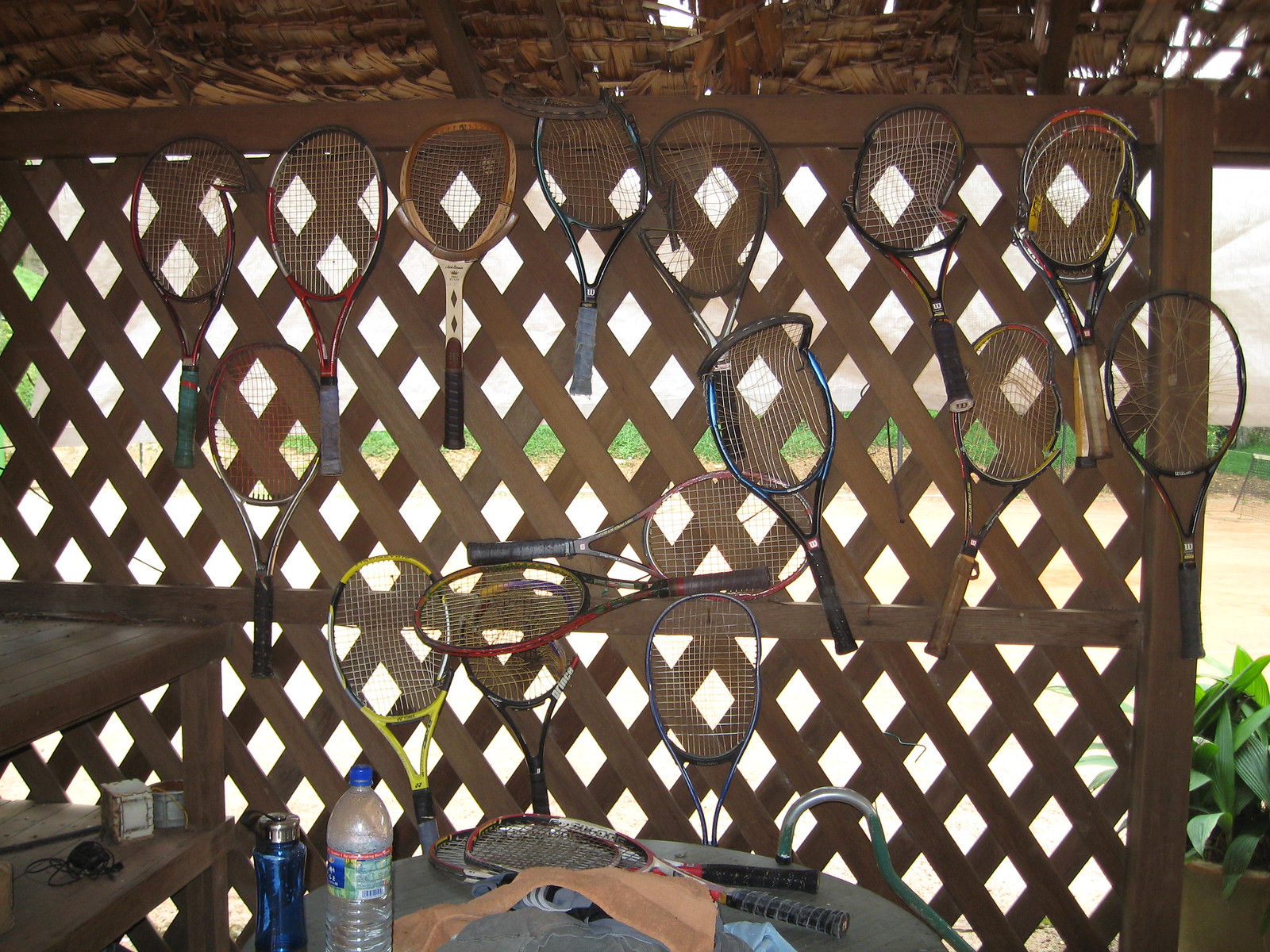This detailed photograph captures an outdoor lattice structure, likely a cabana or shed, with distinctive diamond-patterned wooden lattice walls and a partially decayed thatched roof. The lattice wall, through which light filters in, is adorned with approximately 17 varied tennis rackets. These rackets exhibit a spectrum of colors including blue, red, yellow, orange, white, among others, and vary in condition, with some appearing broken or bent, likely from prolonged use or mishandling.

At the upper section of the wall, a line of tennis rackets is neatly hung, all facing upwards, while in the middle section, rackets are placed more haphazardly, facing various directions. In the foreground, a wooden table is covered with a few more tennis rackets, a grey tube, and a couple of bottles—a translucent plastic bottle with a blue cap and multicolored label, and a smaller reusable blue bottle with a grey cork. A walking cane leans against the table, adding to the miscellany.

To the left of the table, wooden shelving holds additional, less discernible items, including a possibly wooden object with a whitish face. The right side of the image showcases a large plant in a planter just beyond the lattice structure. Through the lattice gaps, a blend of green grass and surrounding fields is visible, with additional greenery lining the background, adding a touch of natural beauty to the scene.